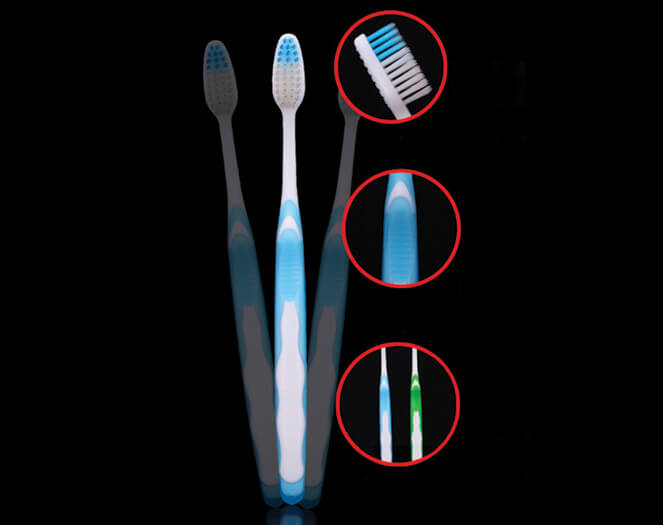The image features a centrally positioned blue and white toothbrush against an entirely black background. The toothbrush, illuminated to highlight its details, displays shadows on both its left and right sides, creating mirror-like images. The toothbrush's design includes a top section of blue bristles and a lower section of white bristles. The upper part of the handle is blue, transitioning to white towards the lower part, with blue accents where the thumb grips the handle.

Three red circles are aligned vertically to the right of the toothbrush, each providing a magnified view of specific parts of the toothbrush. The top circle showcases a close-up of the bristles, emphasizing the dual-color arrangement. The middle circle zooms in on the area where the thumb rests, detailing the blue grip section. The bottom circle offers a view of the toothbrush's backside.